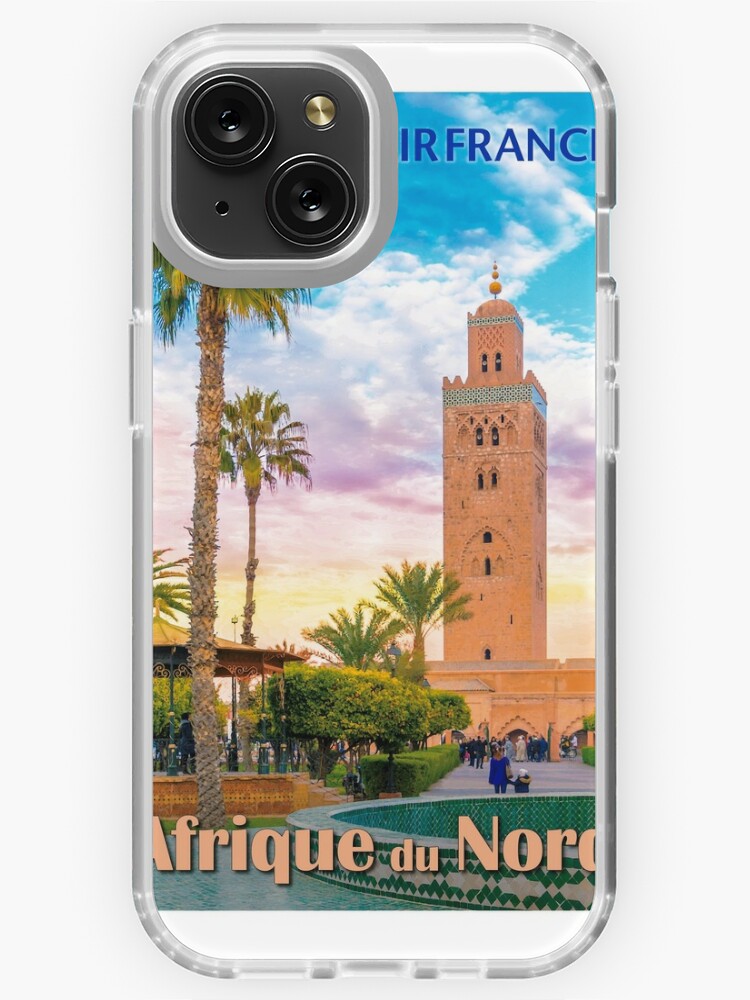This vertical rectangular image depicts the back of an iPhone featuring a cell phone case with a distinct illustration. The case appears to be made of clear plastic, allowing the artwork, likely inserted into the back, to be prominently displayed. The illustration captures a scene from North Africa, as denoted by the partially visible French inscription "Afrique du Nord" at the bottom of the image.

The focal point of the artwork is a large, cathedral-style building or mosque with a distinctive tower shape. The foreground is adorned with several palm trees, including one tall tree that extends into the camera lenses area of the phone. There's a teal and white marble fountain positioned in a courtyard, surrounded by gardens and pathways on either side.

Among these elements, people can be seen walking about, adding life to the scene. At the top of the case, there appears to be the text "Air France," possibly suggesting a thematic connection to travel. The left side of the illustration features another building, corroborating the sense of an urban landscape. This artistic, poster-like design on the back of the phone case blended with the transparency of the frame provides a vivid cultural snapshot, accentuating both the device and its aesthetic cover.